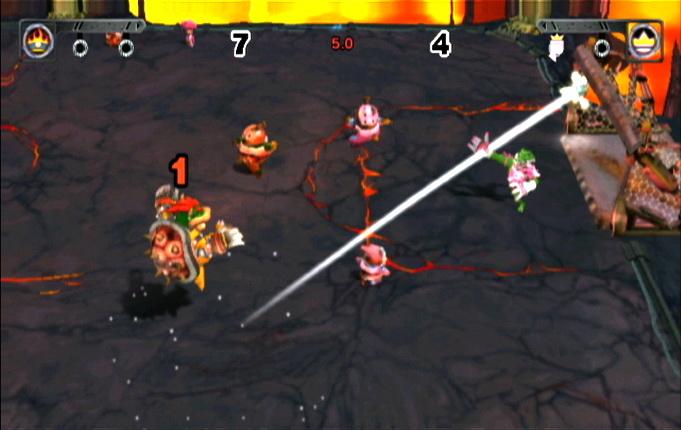The image depicts a vibrant scene from a video game, likely a soccer-themed match set in a fantastical environment. Central to the image are five characters, with one particularly large character that appears to be a boss, reminiscent of a Mario boss. This large character is marked with the number "1," and the top of the screen displays the numbers "7" and "4," possibly indicating scores or levels.

The backdrop is dramatic, featuring a fiery landscape with cracked, blackened lava, creating an intense atmosphere. A beam extends from one character towards what looks like a goal post situated near the large turtle-like boss, indicating some form of objective or interaction.

At the top left and top right corners, various symbols are displayed, adding to the complexity of the game's interface. This scene suggests an imaginative take on a soccer game, infused with elements typical of action-adventure video games, and is being played on a computer.